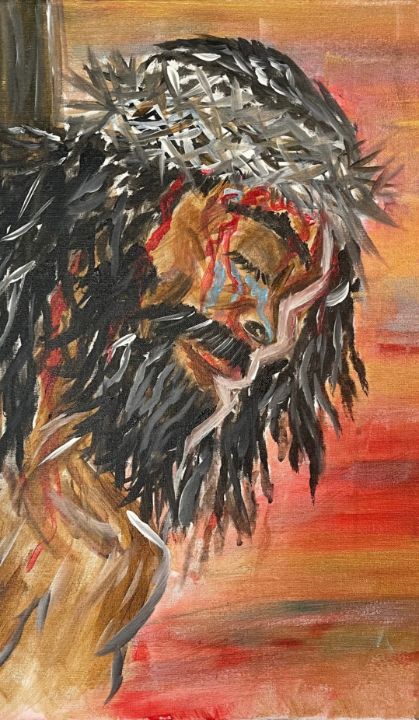This portrait-oriented pastel chalk drawing depicts a semi-abstract image of Jesus Christ, focusing on his upper body. The subject is shown in profile, with his head bent downwards in a serene expression and his eyes closed. He has long black hair, a black beard, and a mustache. Notably, Jesus wears a crown of thorns, from which blood flows down his forehead, creating red streaks along his face. The top of his hair appears gray, transitioning to black further down. His face and chest, portrayed till mid-chest, are a bronze color. To the left, the dark brown wood of the cross is visible. The background is composed of horizontal lines in shades of red, yellow, orange, beige, and hints of blue, contributing to the abstract nature of the artwork. The combined elements of the composition evoke a poignant and reverent representation of Christ on the cross.